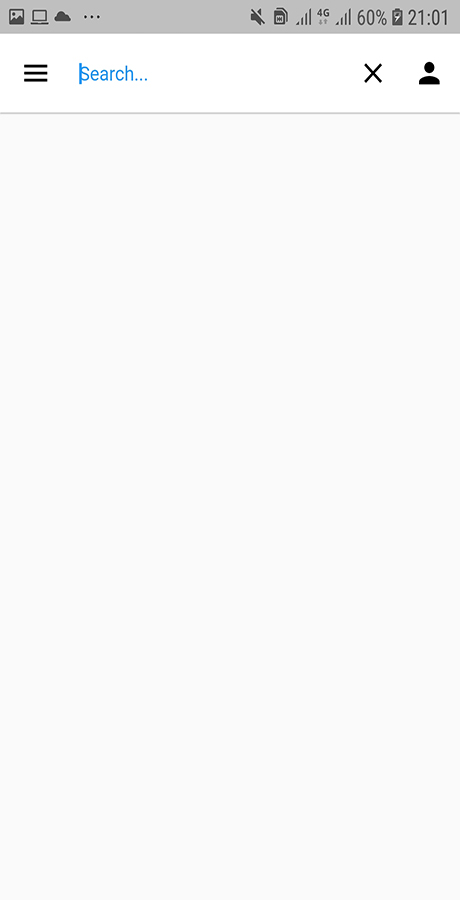This image appears to be a screenshot captured from a cellular phone, with a rectangular shape that is taller than it is wide. At the very top, the image features a small gray status bar running horizontally. Within this bar, there is a sequence of icons including a picture icon resembling a landscape, a laptop icon, a cloud icon, an icon of three horizontal dots, and a speaker icon with a line through it, indicating mute. Additionally, there's a small gray square icon, followed by a signal bar icon which looks like a triangle pointing left to right, and a 4G indicator, a signal strength icon, and a battery icon displaying 60%. There is also a time stamp showing 2101 in military time.

Below the status bar, there is a white search bar with three horizontal lines. The text "search..." is displayed in blue, followed by a black X, and an icon representing a silhouette of a person or a stick figure. Below the search bar is a horizontal gray line. The predominant portion of the image is a large, empty space filled with a light gray or possibly light blue color, with no additional text or visual elements present. The image gives an impression of a minimalistic interface or a blank screen.